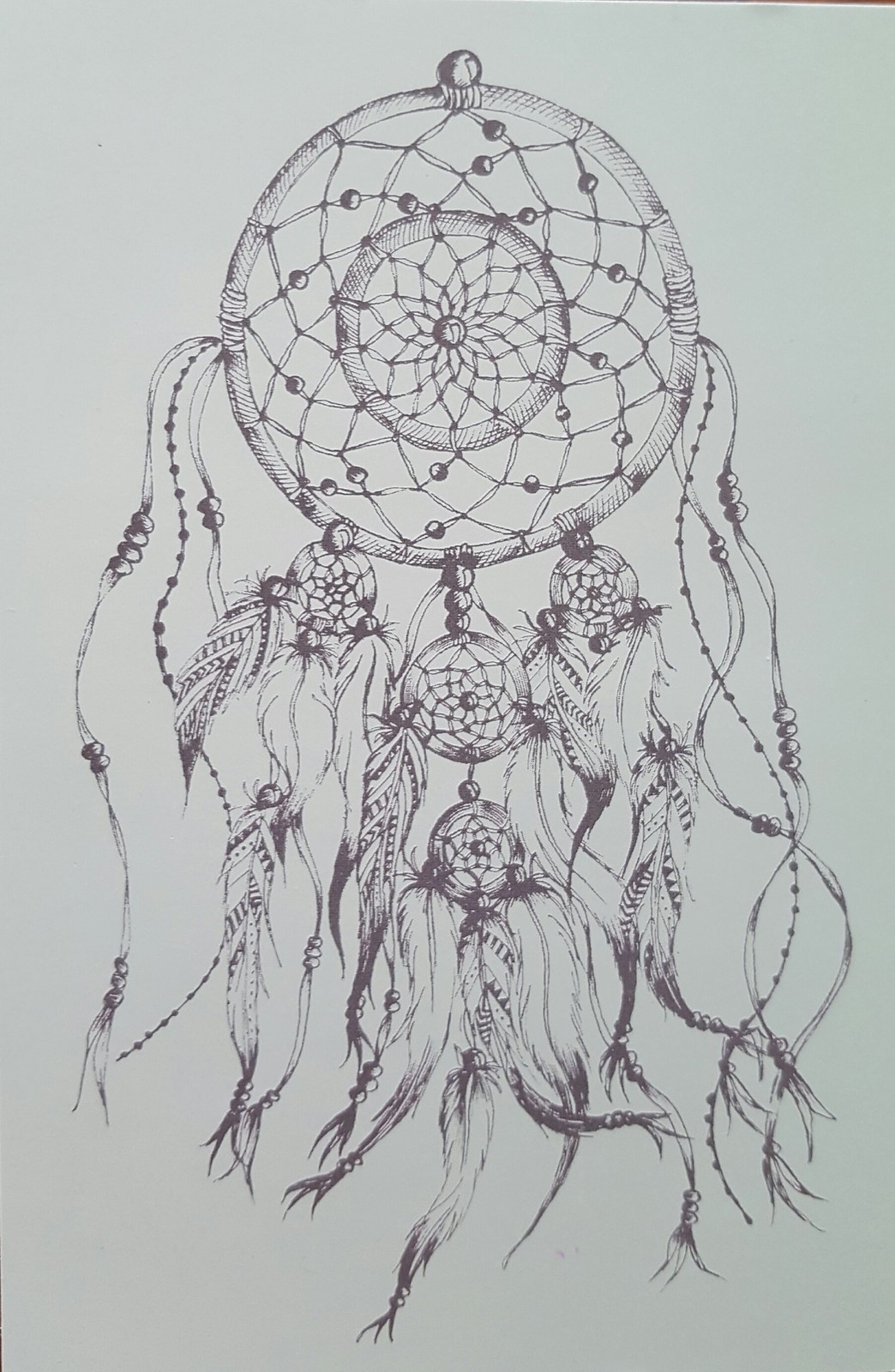This is a detailed sketch of a Native American dreamcatcher, intricately crafted in black and gray shades on a light gray background. At the top of the composition is a large circular frame, woven with crisscross patterns of threads forming a mesh-like design that echoes the shape of a flower. Within this main circle, smaller circular objects and medallions are interspersed, each connected by a series of curvy, twisted tendrils and ribbons hanging downwards.

These descending elements are adorned with tribal beads, feathers, and circular designs. Notably, there are four smaller dreamcatcher-like circles among the hanging structures, positioned with two in the center, one to the left, and one to the right. These smaller circles also feature flower patterns within them, enhancing the overall intricate design. 

The dreamcatcher’s tendrils and ribbons culminate in an assembly of pheasant feathers and artistically designed beads, creating a visually striking balance of nature and craftsmanship. The distinct lack of color in this grayscale depiction accentuates the detailed lines and shaded textures, giving the dreamcatcher a timeless and ethereal quality.